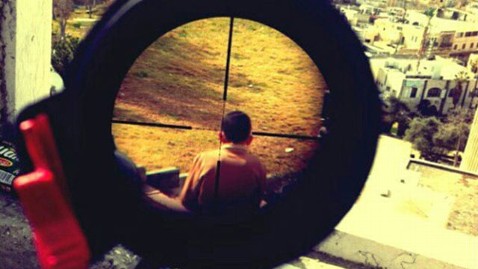The image captures a grim and intense scene through the lens of a rifle scope. At the center of the black-colored scope, marked by precise crosshairs, the focus is on the left side of a person's head, adorned with short black hair and wearing a tan-colored shirt. The view suggests the person is about to be targeted. Surrounding the individual, the background reveals a subtle light yellow hue that contrasts with the dark interior of the scope. The scene is set in what appears to be a Middle Eastern urban environment, characterized by geometric, concrete, and mortar buildings concentrated on the right side of the image. There is also a noticeable red switch or piece of plastic located at the bottom left of the frame, adding to the ominous atmosphere. The perspective of the image implies a high vantage point, possibly from a stone or concrete structure, looking down upon the target with a high degree of zoom, further emphasizing the distance and isolation within the frame.